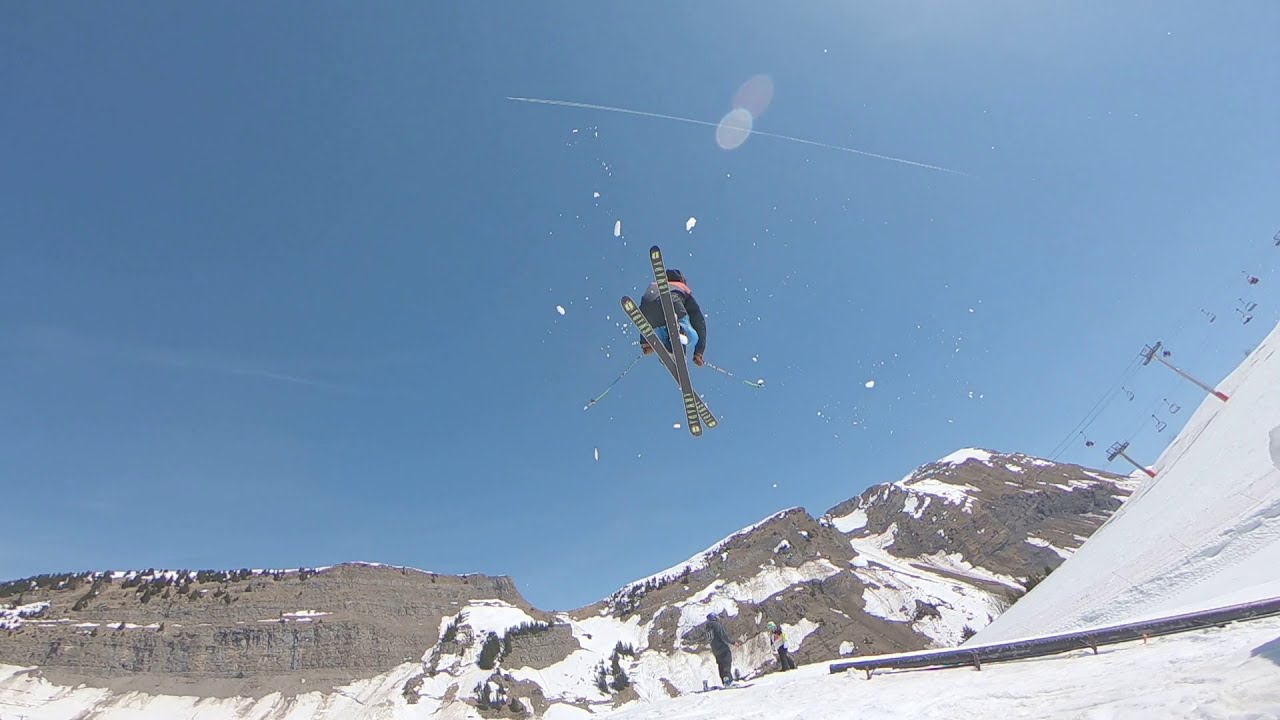The image captures a dynamic scene of a skier caught mid-air during a jump, viewed from the ground looking up. The skier, exhibiting a confident pose, has their knees bent close to their body, strapped into black skis with an indistinct yellow logo. The skier is dressed in a black jacket that features red shoulders and a hood, paired with light blue pants and black and red gloves. They also wear a black beanie. The skier's poles are splayed outward to the left and right.

Beneath the skier, the ground is covered in snow, and a dark track wall or some other structure is visible. To the right side of the image, a ski lift is seen transporting people up the mountain. The background showcases a picturesque landscape with steep, snowy hills and towering mountains. One conspicuous mountain on the left is covered in dark gray rocks, while the central mountain has a snowy peak. The photograph appears to be taken with a fisheye lens, adding a subtle distortion that curves the image slightly, giving a wider field of view. The clear, daytime sky, high sun, and tiny figures on the ski lifts all contribute to the vibrant, energetic scene of this ski resort.